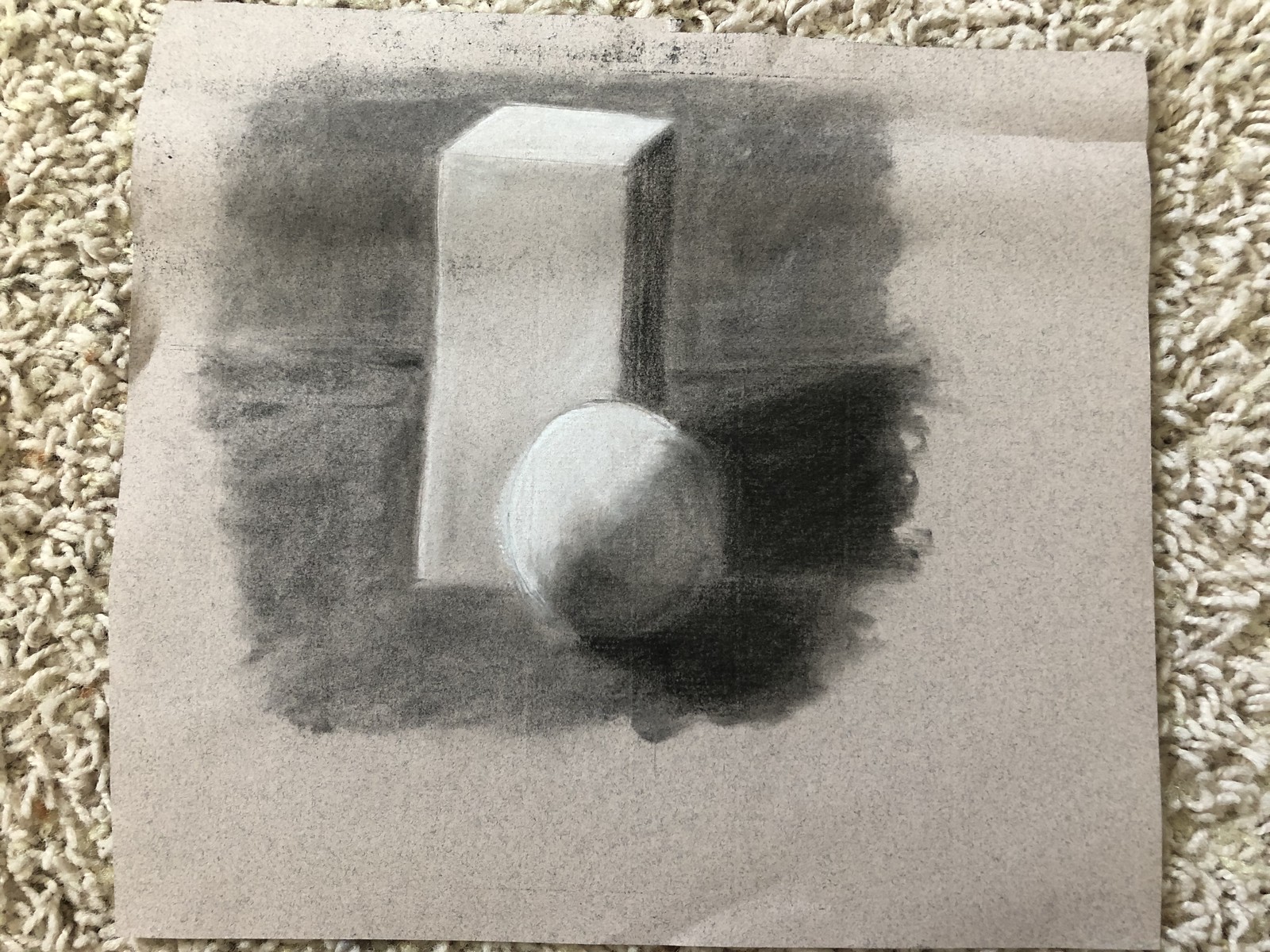This image captures a meticulously drawn geometric composition featuring a metallic silver cube and sphere. The drawing is rendered on a brownish-gray sheet of what appears to be construction paper. The paper is resting on a light-colored, loose-threaded carpet. The background of the drawing includes a predominantly gray square with an area of black shading near the bottom, creating a subtle depth effect behind the cube and sphere. The overall setting suggests an informal, creative workspace, with the detailed geometric design standing out against the textured and muted backdrop of the carpet and construction paper.